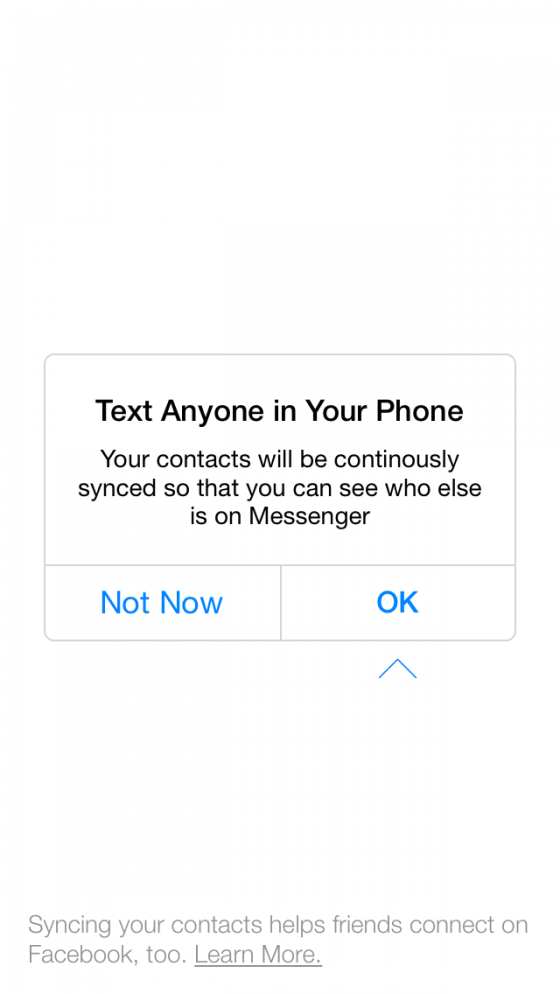The image depicts a notification pop-up on an iPhone, resembling the interface typically seen in the settings menu. This box features a clean white background bordered by a gray outline. At the bottom of the box, two gray lines form a "T" shape, with one line running horizontally across the width and the other vertically bisecting the horizontal line.

At the top, bold black text reads, "Text anyone in your phone." Below this, in non-bold black text, the message continues on multiple lines: "Your contacts will be continuously synced so that you can see who else is on Messenger."

The lower section of the pop-up presents two clickable options divided by the "T" shape: "Not now" on the left, written in blue with the letters "N" and "OW" capitalized, and "OK" on the right, also in blue with both letters capitalized. 

Beneath these options, the text in smaller font states, "Syncing your contacts helps friends connect on Facebook too." An arrow pointing upward in blue highlights the "OK" button. At the very bottom, a "Learn More" link is provided for additional information.